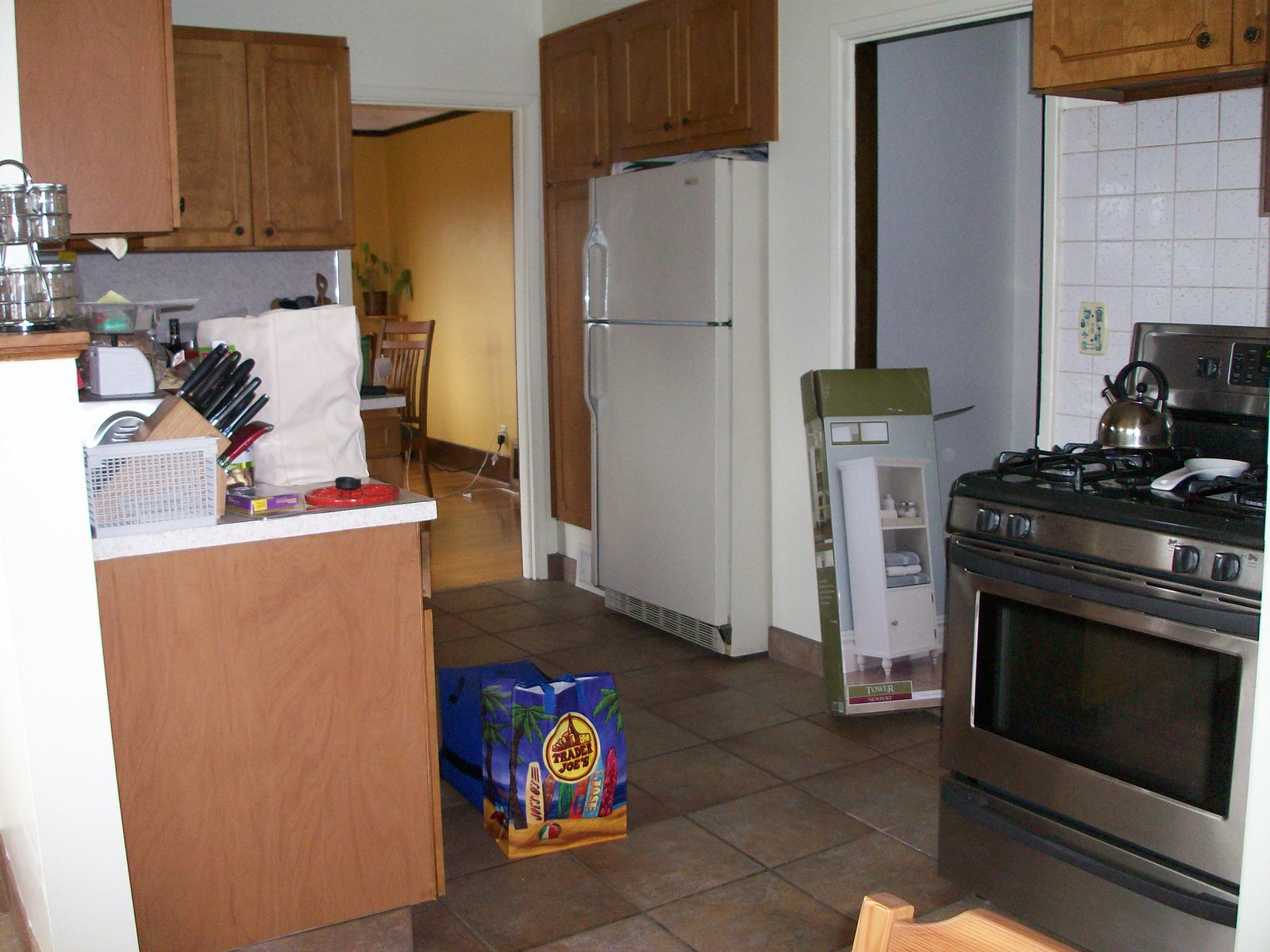The photograph captures a well-organized kitchen within a house, presenting a blend of contemporary and traditional elements. On the right side of the image, there's a sleek stainless steel all-in-one gas cooktop with an oven underneath, accompanied by a drawer beneath the oven. The stove is backed by white square ceramic tiles, which extend to the bottom of an overhead cabinet, creating a crisp, clean backdrop.

Adjacent to the stove, there is a door framed in white, flanked by a white wall. Behind this door, a hint of gray is visible, suggesting a different room or storage area. Leaning against the doorway is a box featuring an image of a bathroom cabinet designed for towels and decorative items.

To the left of the door stands a white refrigerator, which is encased in oak cabinetry on its top and left sides, seamlessly integrating it into the kitchen's layout. The kitchen floor is adorned with dark square ceramic tiles, providing a sturdy and stylish foundation.

On the left side of this galley-style kitchen, additional cabinets and countertops line the wall. The countertops appear to be made of Formica, offering a practical and durable surface for kitchen tasks. A set of knives is neatly arranged on the counter, emphasizing the kitchen’s readiness for meal preparation. Above these countertops, more cabinets provide ample storage, completing the functional and aesthetic design of the kitchen.